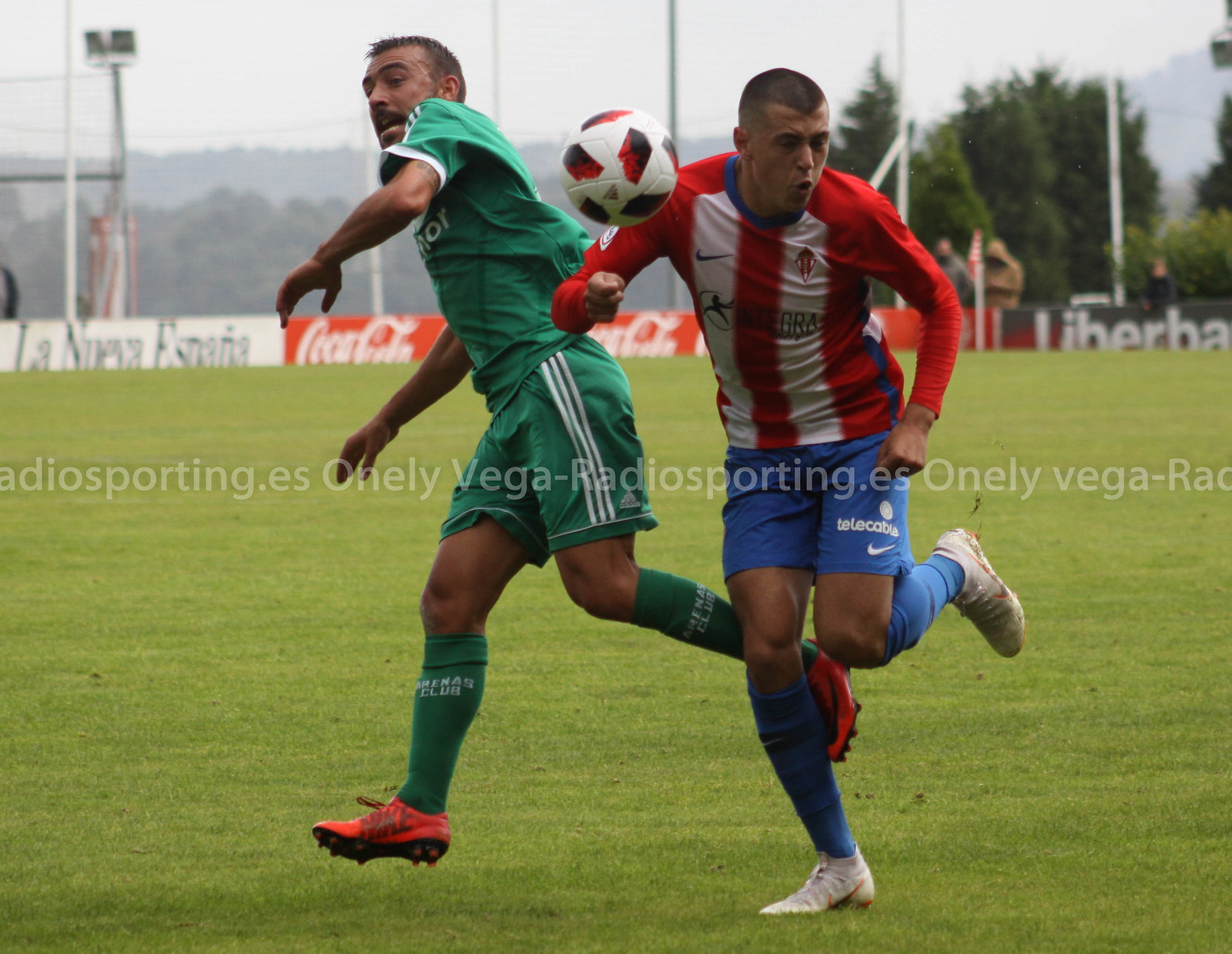The image captures two soccer players in mid-action on a green grass sports field, both attempting to gain control of a red and white soccer ball suspended in the air. The player on the right is dressed in blue shorts, blue socks, gray shoes, and a red long-sleeve shirt featuring two vertical white stripes and the "Integra" branding on the chest. The player on the left sports green shorts, green socks, and a green shirt with white stripes, complemented by red Nike cleats. In the backdrop, a white and red wall adorned with various brandings including "Coca-Cola," "La Nueva Estarnia," "La Berba," and "radiosporting.es" is visible. The wall stands against a hazy day, with stadium lights overhead and large trees in the distance adding depth to the scene.